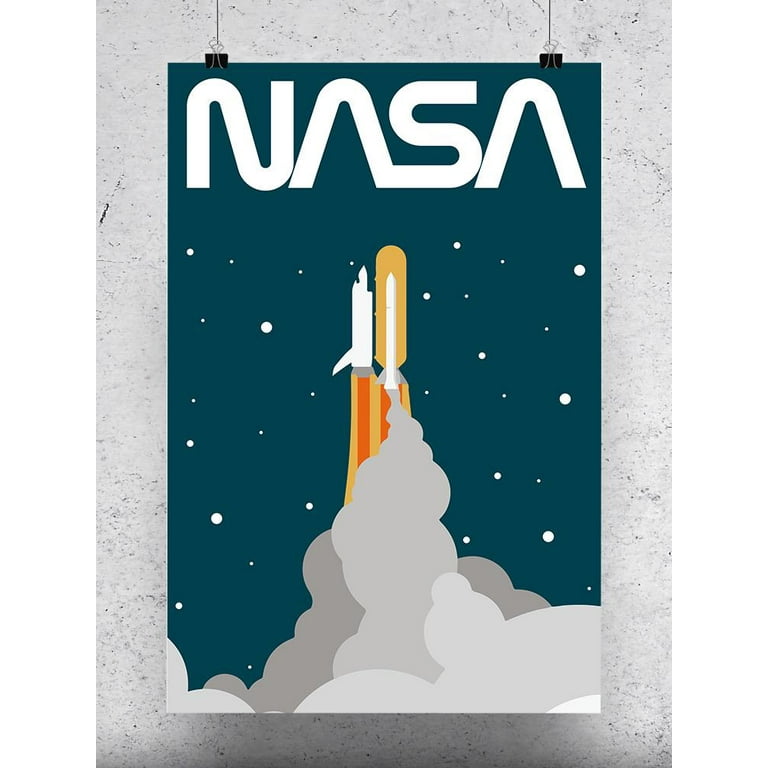This image is a detailed artistic representation of a NASA poster, prominently hung against a gray background speckled with black spots. At the top of the dark blue section of the poster, "NASA" is written in a distinctive, stylized font where the A’s are designed like upside-down V's without the middle line. The central focus of the artwork is a conceptual rocket, displaying a dynamic white and yellow color scheme. The rocket is depicted with a yellow propulsion container, and its bottom emits vivid jets of orange and yellow flames. Below the flames, thick plumes of white, gray, and dark gray smoke, illustrated in blocky, unblended shapes, billow downward. The dark blue background of the image is dotted with variously-sized white circles, representing stars, enhancing the cosmic theme of the drawing clipped to the grayish patterned backdrop using two black binder clips.